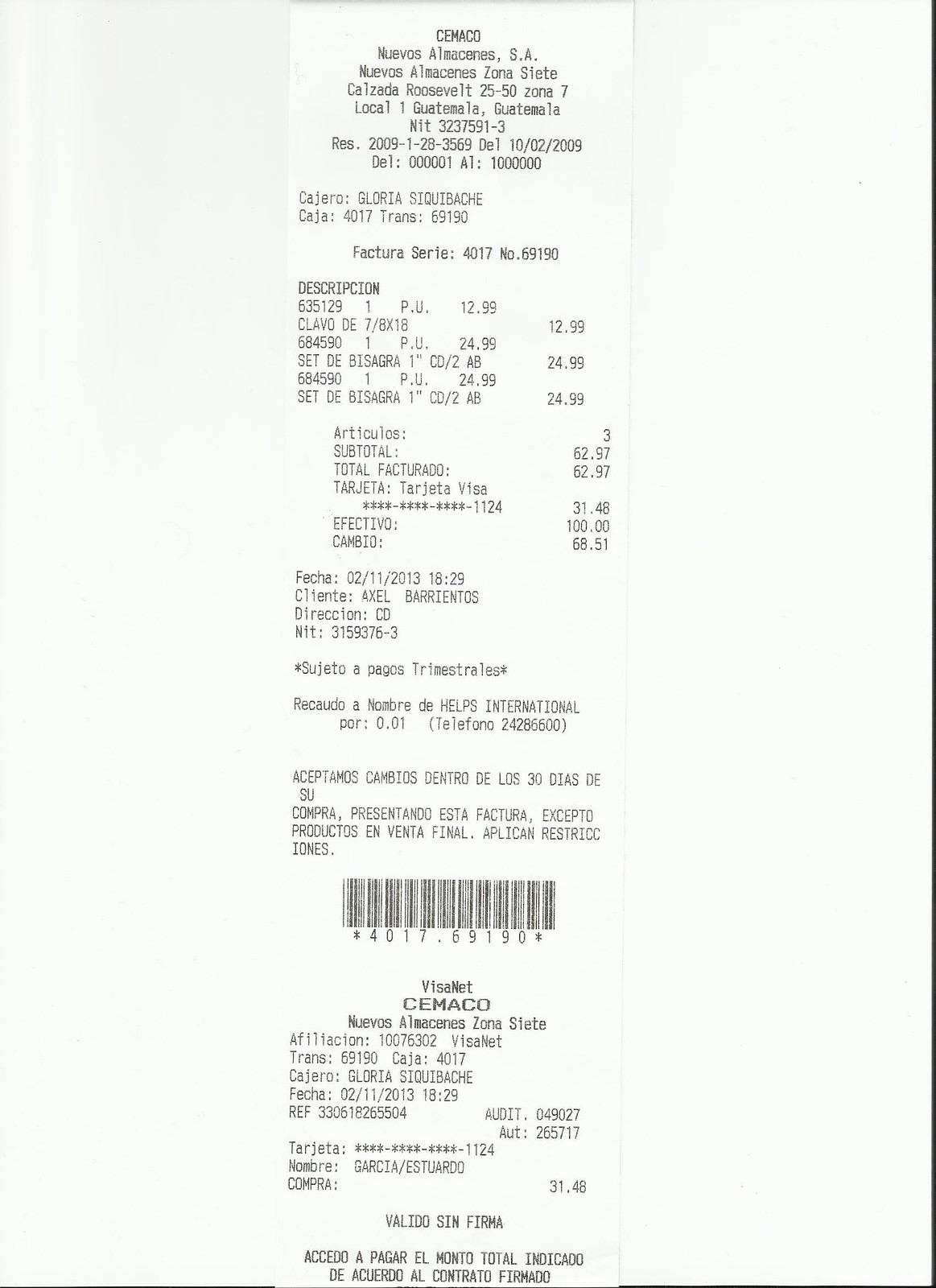This image shows a detailed scanned receipt from a store called Cemaco, prominently displaying text mostly in Spanish. At the top, the receipt includes the store's name, "Nuevos Almacenes, S.A.," along with its address: "Nuevos Almacenes, Zona 7, Calzada Roosevelt, 25-50 Zona 7, Local 1, Guatemala, Guatemala." Beneath this, there is the NIT number "3237591-3" and various other numerical details, including "R.I.S. 2009 1 28 3 5 6 9," and "D.E.L. 10-02-2009." Another section includes a distinctive barcode in the middle, labeled "401769190 star." The customer's name is noted as Possible Ecoloria, and the cashier is identified as Gloria Siquibache. The subtotal of purchased items amounts to 6297, although another mentioned total is 6851. The receipt is filled with many words and numbers in Spanish, detailing the purchase transaction extensively.